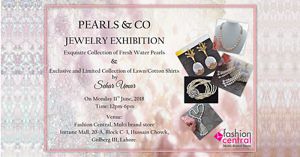The image is a detailed advertisement for a jewelry exhibition by Pearls & Co., set against a visually rich background featuring a repeating pattern of diamonds, pinkish and teal hues, and a pink, floral design. At the very top center, bold black text reads "Pearls & Co." followed closely by "Jewelry Exhibition." Although much of the text is small and challenging to decipher, it contains essential information about the exhibition dates and venue details. The right side of the advertisement displays an assortment of jewelry—earrings, necklaces, a bracelet, and possibly a keychain—organized within individual squares arranged in a cascading pattern. Among the jewelry pieces are pineapple earrings, dangling earrings, and a pearl necklace. The entire layout is framed within a pink square that borders the text and images. In the bottom right corner, a small pink diamond symbol and adjacent text indicate affiliation with Fashion Central.